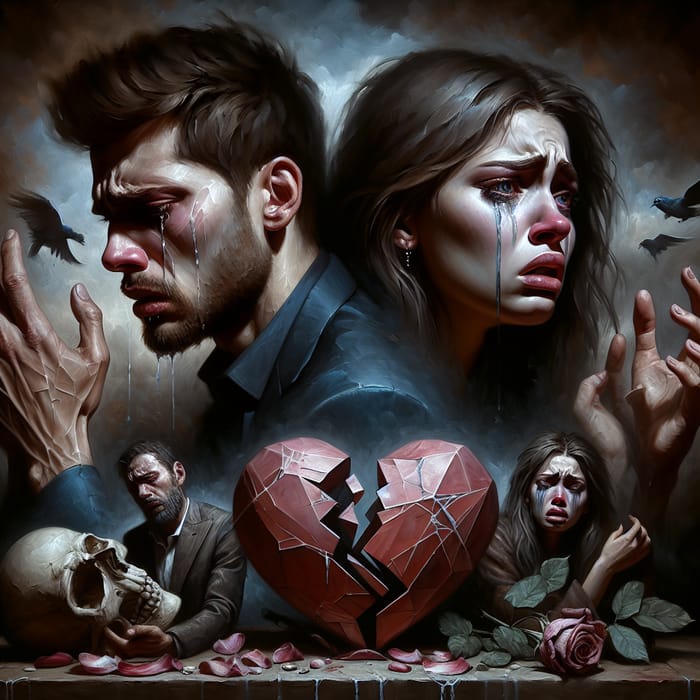Against a dark, stormy backdrop filled with gray and black clouds, an A.I.-generated image captures an intense scene of heartbreak. In the center of the composition, a young man and woman stand back-to-back, dark-haired and in deep sorrow. Prominent tears stream down their faces. The woman, adorned with earrings and holding her hands to her face, cries literal blue paint that contrasts sharply with her bright red nose. Her male counterpart on the left, clad in a blackish-gray and blue suit, is depicted with tears and a startling image where his temple appears to be crying out the side of his brain. Below them, a large, red, cracked-in-half heart is prominently displayed, signifying profound emotional pain. Scattered broken pieces of the heart litter the table beneath them. To the right, another woman, also shedding blue painted tears, holds her hands to her face. At the bottom center, a man sorrowfully caresses a gigantic skull. All around, black birds fly ominously, heightening the sense of devastation and despair in this surreal, heart-wrenching scene.